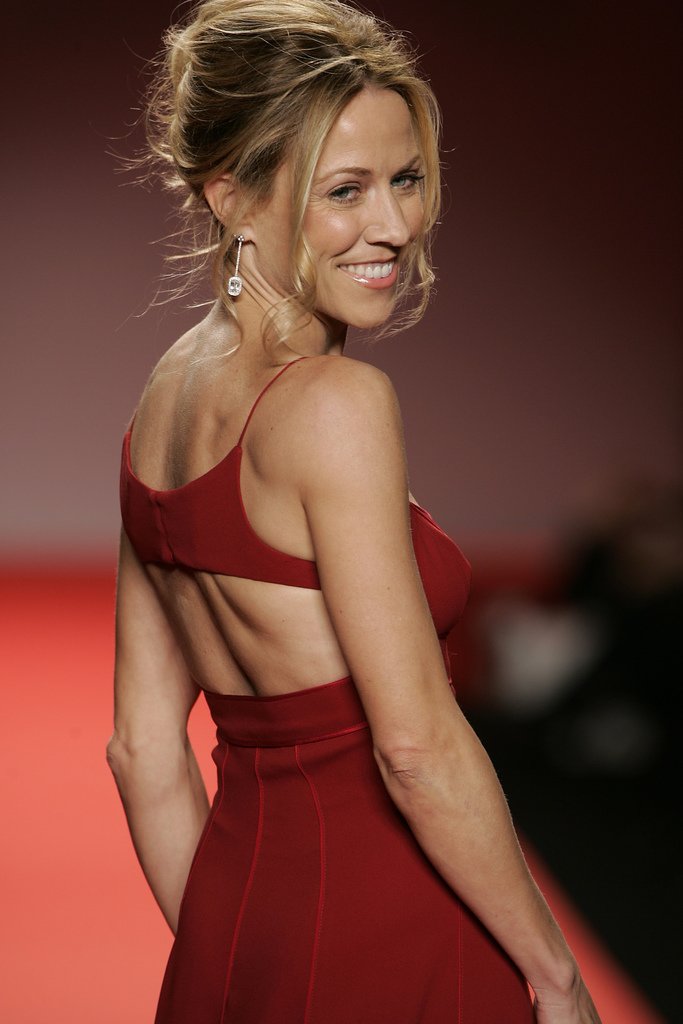This highly-stylized, professional-grade photograph showcases a sophisticated classic model shot featuring a very attractive Caucasian woman with blonde hair. She is centrally positioned, facing away from the camera but angled slightly to look over her right shoulder with a captivating smile. Her professionally styled makeup complements her long blonde hair, which is swept back and gathered into an elegant updo at the crown of her head, with wisps gently framing her face. She wears long, dangling earrings that add to her glamorous appearance.

She is adorned in a striking red halter-style dress, which cinches tightly at her waist before flaring out over her hips. The back of the dress is notable for its narrow strapping that elegantly crosses her bare shoulder blades, leaving her arms and the midriff of her back exposed. Her relaxed stance, with arms loosely bent at the elbows, exudes confidence and poise.

The setting of the photograph suggests a red-carpeted runway, albeit blurred to keep the focus firmly on the model. The background extends from the midline of the photograph upward in a heavily filtered red or maroon hue, perhaps indicative of a stage. On the right edge of the image, there appear to be spectators seated along the side of the red carpet, adding to the ambiance of a high-profile event. The combination of her radiant smile, poised posture, and the elegant setting creates an image that is both timeless and captivating.